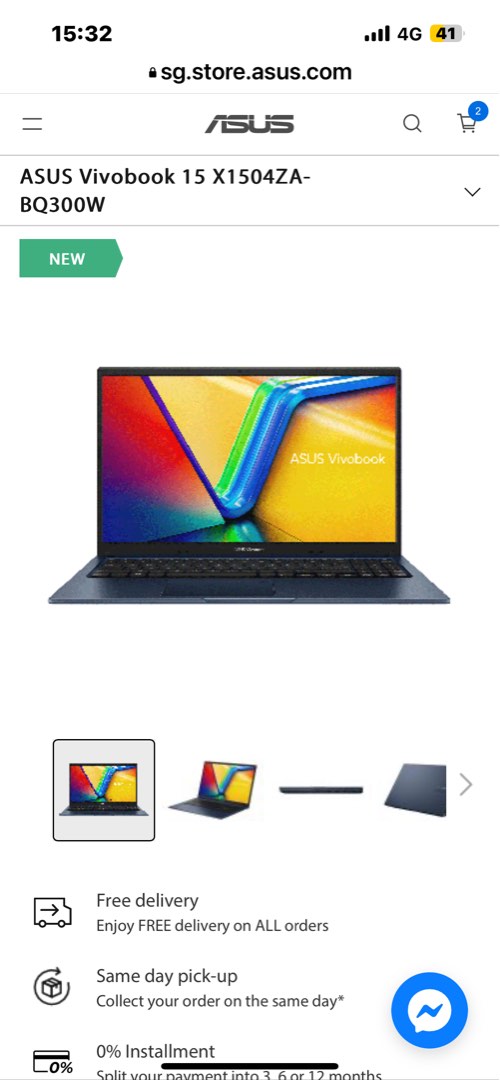The image features a smartphone displaying the website sgstore.asys.com. The phone's battery life is shown as 41%, shaded in gold, and it is connected to a strong 4G network. The time displayed on the phone is 15:32. Beneath the website address is the ASUS logo, which is prominently featured.

The site appears to be advertising an ASUS VivoBook, including its model number. A green icon or bar labeled "NEW" in white text is visible, highlighting the latest product. The main section of the page showcases a colorful image of the ASUS VivoBook, incorporating hues of gold, green, blue, and red. The image includes a detailed view of the keyboard and various angles of the laptop: the side view, front view, folded side view, and a top-down folded view.

The website promotes several key benefits, such as free delivery on all orders, symbolized by a box with an arrow, and same day pickup, indicated by a box with a circle around it and an arrow. Additionally, the site offers 0% installment plans, depicted by a blue circle featuring a smaller white circle with a blue insignia inside. The shopping cart icon shows two items currently in it, and there is also a search bar for easy navigation.